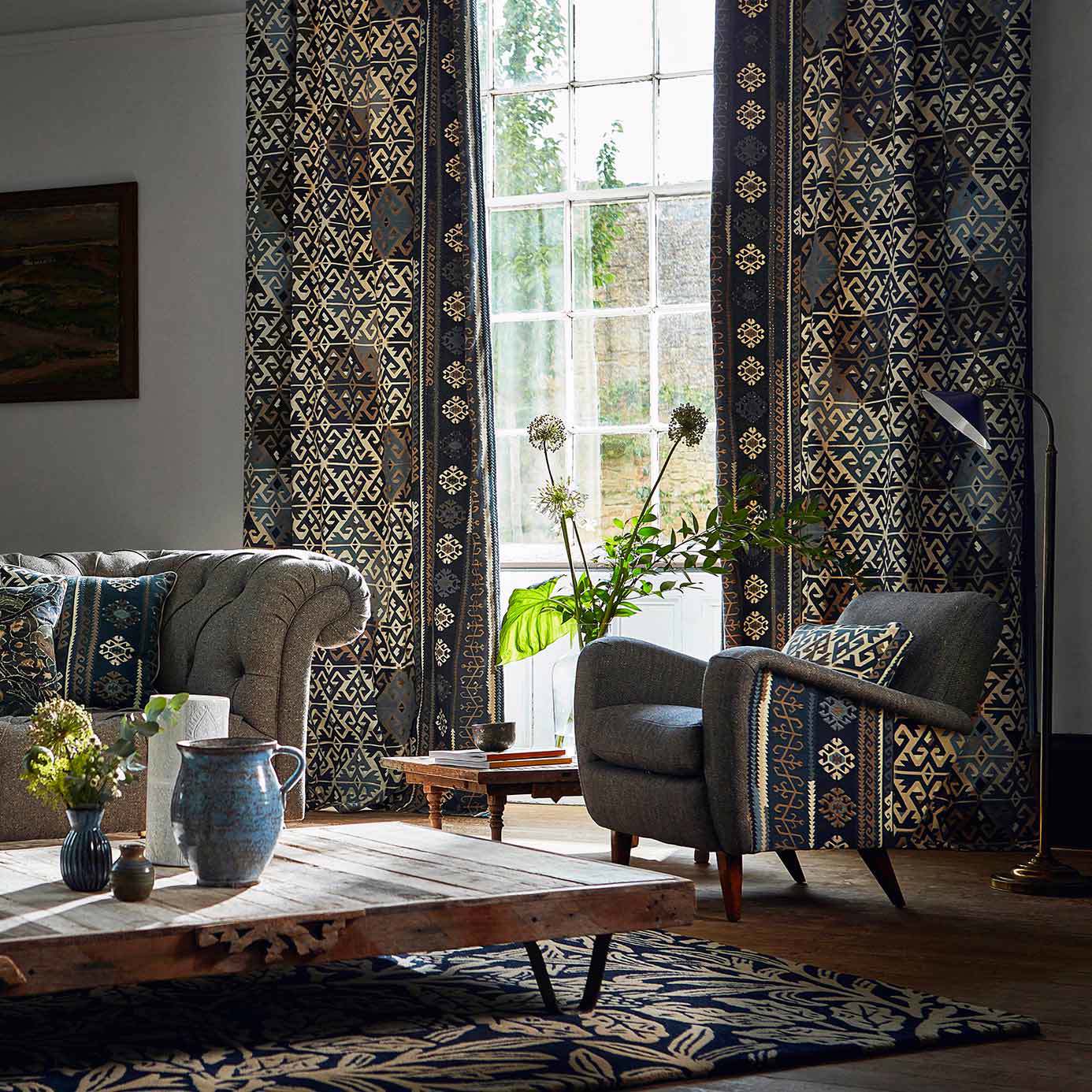The photograph depicts a professionally designed formal living room bathed in daylight. Dominated by a large floor-to-ceiling window with multiple glass panes, the space is adorned with striking curtains featuring a floral pattern and geometric designs in shades of brown, blue, and gray. The medium brown wooden floor is partially covered by a rug with a navy blue background and light tan leaves and flowers. Central to the room is a low-lying coffee table with metal U-shaped legs. It holds a blue vase, a large blue pitcher, a white tall cylinder vase, and a smaller brown jar. To the right of the table is a gray chair with matching geometric pattern cushions, while behind the table stands a gray couch with complementary throw pillows. The walls, painted in a sophisticated gray tone, encase this elegantly appointed living area.